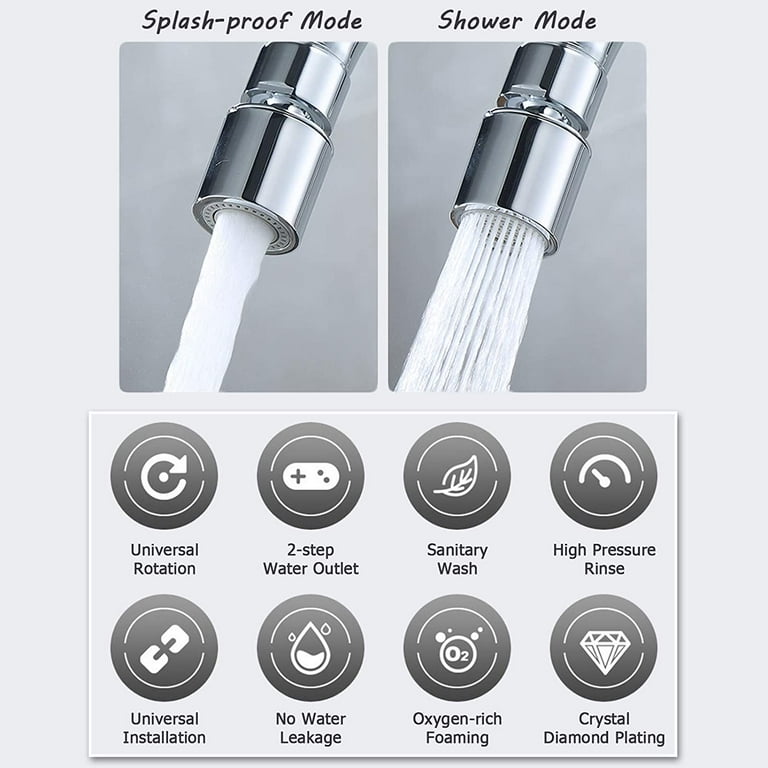The image features a detailed depiction of a kitchen faucet nozzle in a predominantly black-and-white aesthetic, set against a light gray background. At the top are two vertical rectangular photographs placed side by side—the left labeled "Splash Proof Mode" and the right labeled "Shower Mode." The "Splash Proof Mode" image shows the nozzle emitting a solid, cylindrical stream of water, while the "Shower Mode" image depicts the nozzle releasing water in multiple separated jets. Below these pictures is a horizontal rectangular gray box containing two rows of four icons each, accompanied by descriptive text. The top row icons are labeled: "universal rotation," "two-step water outlet," "sanitary wash," and "high-pressure rinse." The bottom row icons are annotated as: "universal installation," "no water leakage," "oxygen-rich foaming," and "crystal diamond plating." Each icon is situated inside a dark gray circle and is represented by distinct graphical symbols such as a circle with arrows, a joystick, a leaf, a gauge, connected squares, a water droplet, bubbles labeled "O2," and a diamond, conveying a variety of functionalities and features of the faucet nozzle.